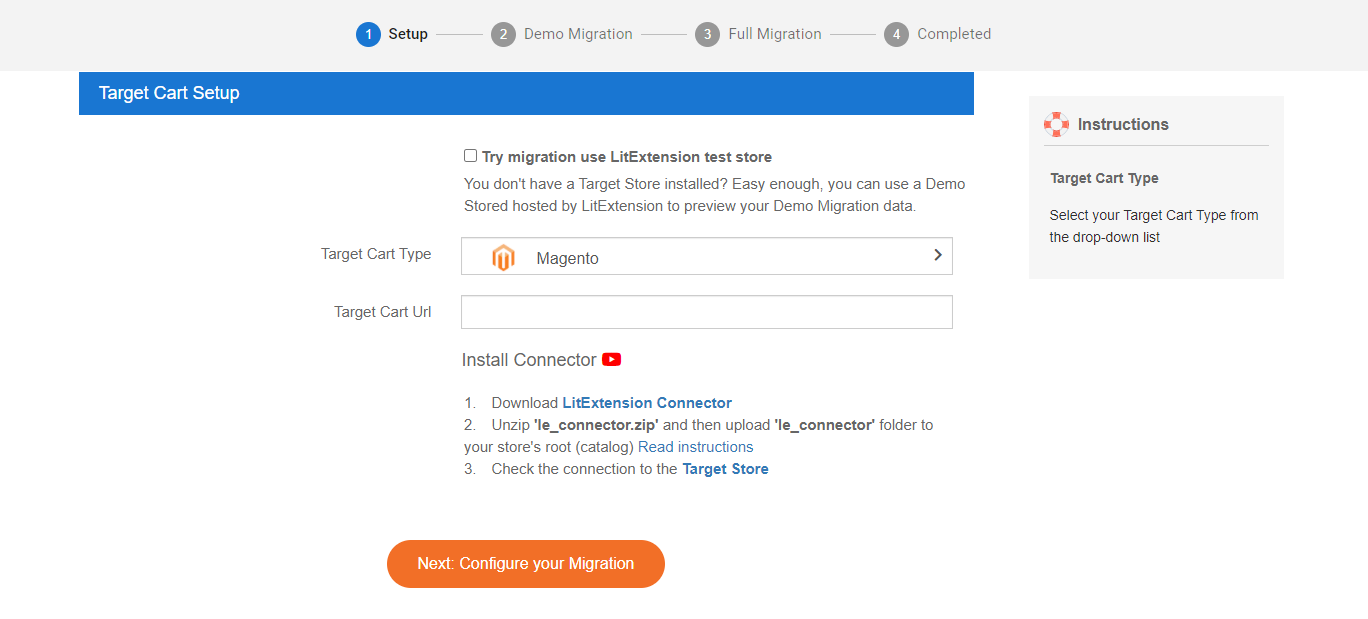The image showcases a horizontally oriented web page with a predominance of white space, especially at the bottom. The layout lacks any left, bottom, or right borders, blending seamlessly into the white background. At the top of the page, there is a pale gray banner that outlines a four-step process. The first step, labeled "Setup," is highlighted, while the subsequent steps—"Demo Migration," "Full Migration," and "Completed"—are grayed out.

Beneath the gray banner is a shorter blue banner containing white text, which reads "Target Cart Setup" on the left-hand side. Adjacent to this, on the right, is a small gray box with instructions: "Target Cart Type. Select your target cart type from the drop-down list."

Centrally aligned and moving downward, there's a prominent section that starts with a box labeled "Try Migration, Use LIT Extension Test Store" with an explanatory text beneath it. Following this, a scroll bar is labeled "Target Cart Type," displaying "Magento" with a right-pointing arrow. Moving further down, there is a field designated for the "Target Cart URL." Towards the bottom of this segment, there is a button labeled "Install Connector," accompanied by a video play button and three instructional steps. At the very bottom, centrally positioned, is an orange oval-shaped button with the text "Next, Configure Your Migration."